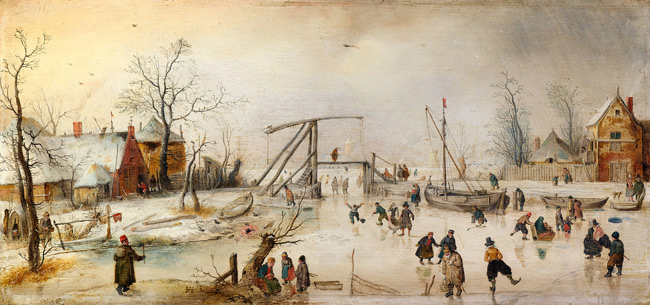This rectangular painting, approximately five inches wide and two inches high, depicts a bustling outdoor winter scene in an old-fashioned town. The top half of the picture features a sky transitioning from pale yellows on the left to cream in the center, and shifting to grays as it reaches the right. Below the sky, the ground is covered in white, portraying a snow-covered landscape.

In the foreground, the center holds a frozen lake where numerous people are ice skating, creating a lively scene filled with men, women, and children enjoying the winter festivities. Some of the skaters are adorned in period clothing such as top hats and trench coats, hinting at a historic setting. Notably, a person in the bottom left corner stands out with a red hat and a brown jacket.

On either side of the painting, light brown wooden buildings with snow-covered rooftops frame the scene. The building on the far right has a distinctive sharp-pitched roof. Trees without leaves, with trunks in brownish-gray tones, dot the landscape alongside the brown and dark brown patches of grassy banks.

Several wooden boats are visible on the frozen lake. One boat, equipped with poles, has a sail and is stuck in the ice, while another smaller, empty rowboat also made of wood can be seen. In the distance, a pier extends into the background, adding depth to the portrayal of this winter wonderland.

Overall, the painting is rich with detail, capturing a moment in time where the townsfolk gather to skate and socialize amidst a rustic, snow-blanketed village.